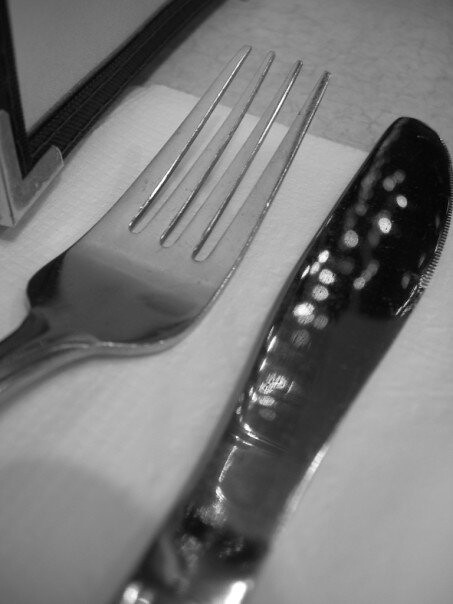A close-up black and white photograph captures a detailed and intimate view of silver utensils set on a tabletop. On the left, the head of a well-used silver fork with slightly raggedy tines is clearly seen. The fork's handle is not visible, indicating the image's focus on the utilitarian elegance of its tines. To the right, a slightly blurry case knife with a dimpled surface reflects small beads of light, giving it a textured appearance. Both utensils rest on a white napkin that sits atop what appears to be a white or gray tablecloth. The upper left corner of the image includes part of a black-framed object with metal detailing that could be a framed picture or a menu, adding an additional layer of context to the overall composition. The photograph's artful use of black and white enhances the textures and contrasts, resulting in a strikingly beautiful and evocative image.